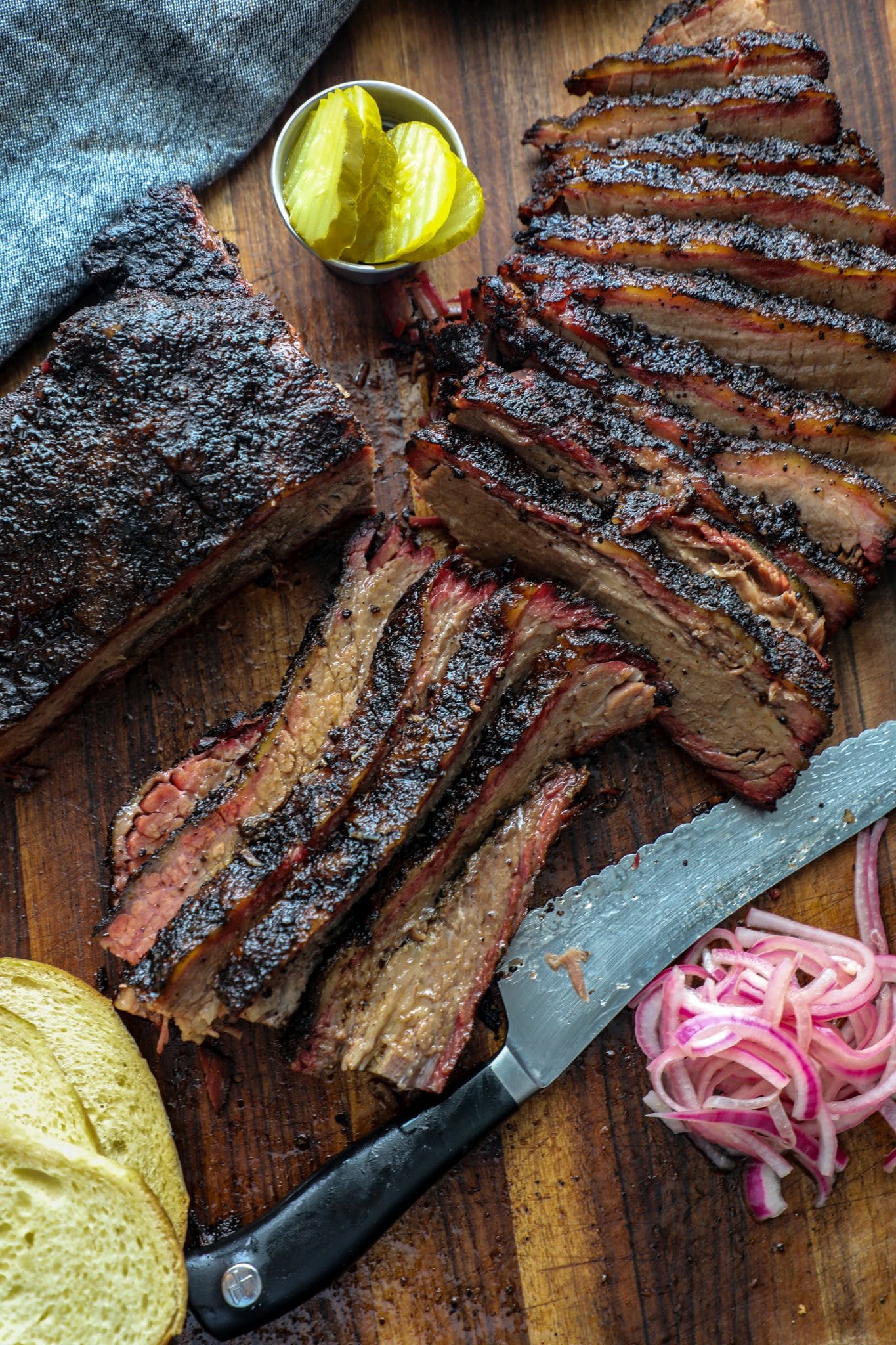The image is a bird's eye view of a rustic, well-used wooden cutting board showcasing a spread of delicious food, likely for a food blog. The centerpiece is a partially cut brisket, with half of it sliced thinly and fanned out, while the other half remains in a hefty, charred chunk. A large serrated knife, seemingly not ideal for the task, is partly hidden under the meat, suggesting a struggle in cutting. Accompanying the brisket, there is a neat stack of two pieces of bread in the bottom left corner, likely intended for sandwiches. The upper left of the image features a small metal dip cup with several slices of pickles. Beside it and slightly below, a modest pile of red onions completes the rustic arrangement.